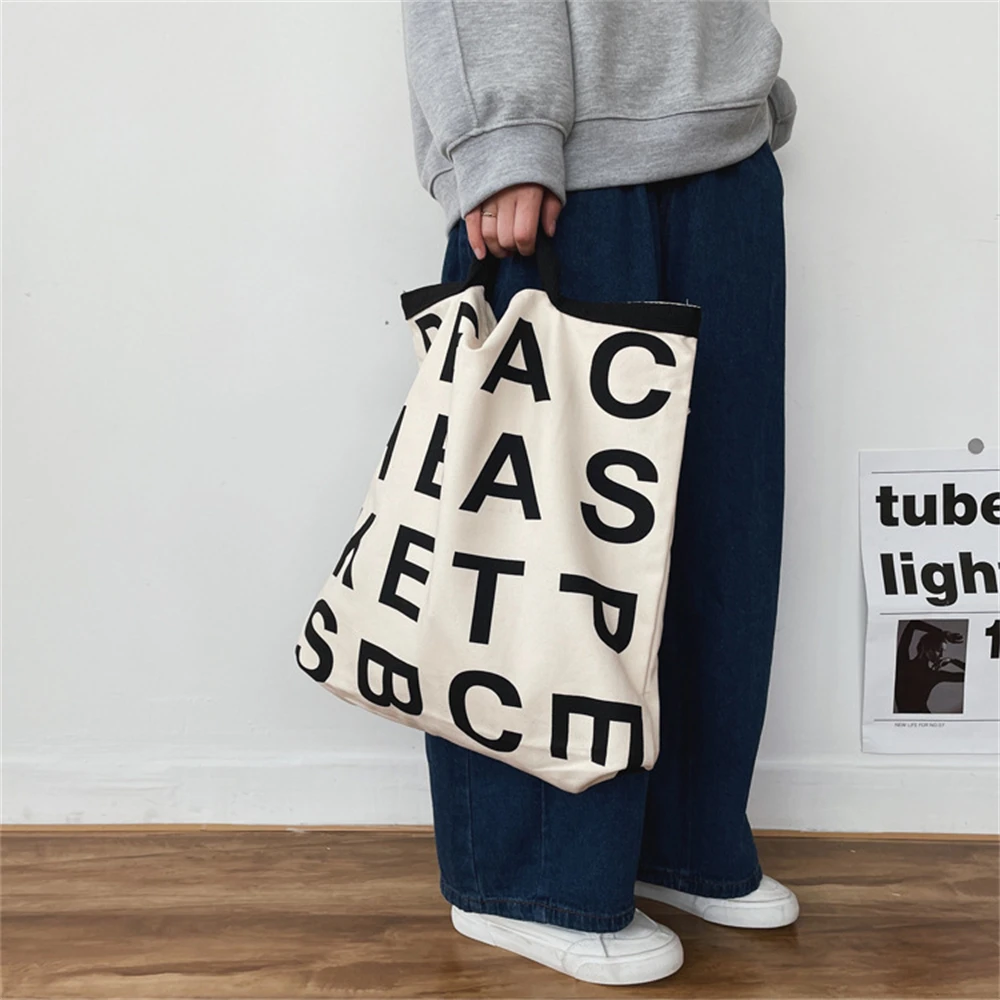The image depicts a person, likely in a promotional setup for a bag, standing on a horizontal-grain brown hardwood floor. The individual is attired in a gray sweatshirt, wide-legged navy blue jeans, and white sneakers. Their right hand, which sports a ring on the ring finger, holds a light-colored canvas bag adorned with a black trim at the top. Black sans serif letters on the bag form partial and fragmented words, including "A C B A S E T P S B C E," with some letters oriented differently. In the background, a white wall with white wooden trim at the bottom features a small sign in the lower right corner displaying the text "Tube L-I-G-H." The person stands facing the right side of the image, with only their lower torso and part of their midsection visible, highlighting the modern and simplistic design of the scene.